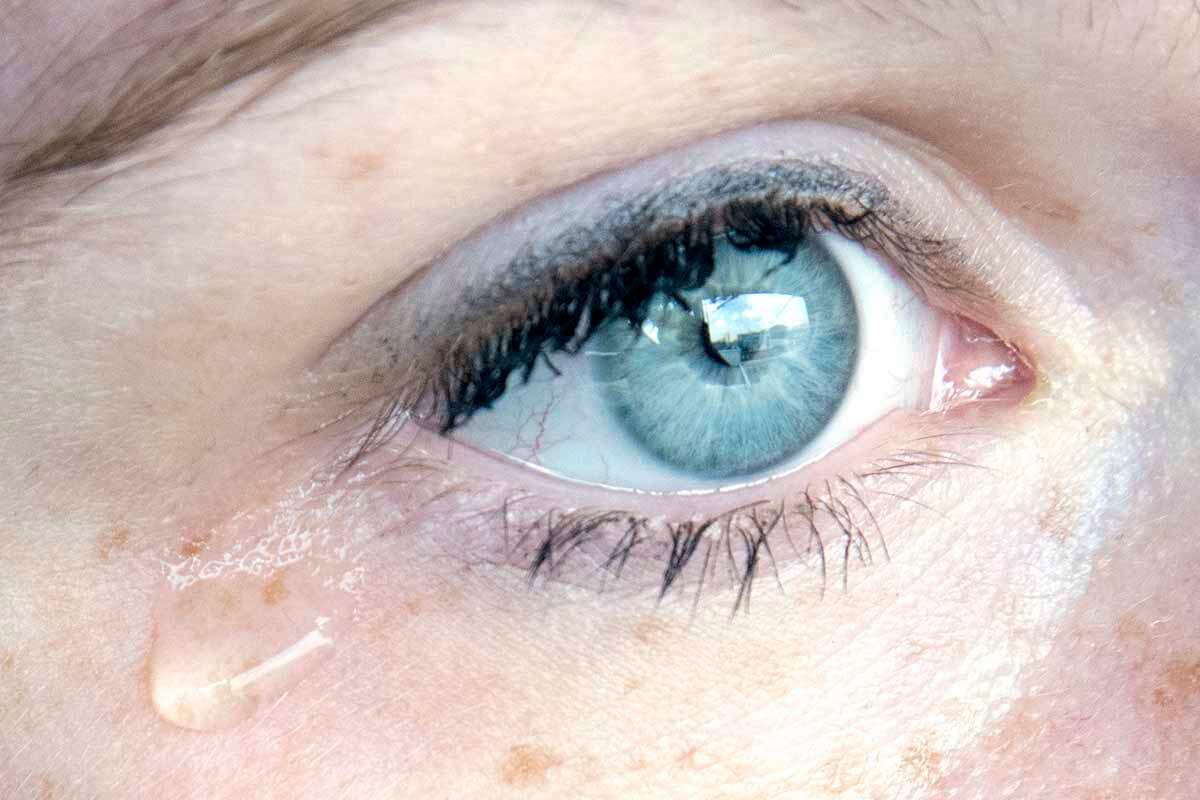This image is an extreme close-up of the left eye of a person, likely a woman judging by the makeup. The eye is strikingly light blue with a bluish line of mascara that complements the iris. The top lashes are heavy with mascara, while the bottom lashes have little to none. Above the eye, strands of brownish-blonde hair can be seen, and a fair-haired eyebrow is partially visible.

The skin around the eye is fair but shows signs of sun damage and minor blemishes, including some brownish-red discoloration and dark markings. The eye has a slight bloodshot appearance, with visible red veins. A single tear is captured rolling down the left side of the person's cheek, evocative of emotion. The detailed focus on the eye and tear gives the image a poignant and intimate feel.